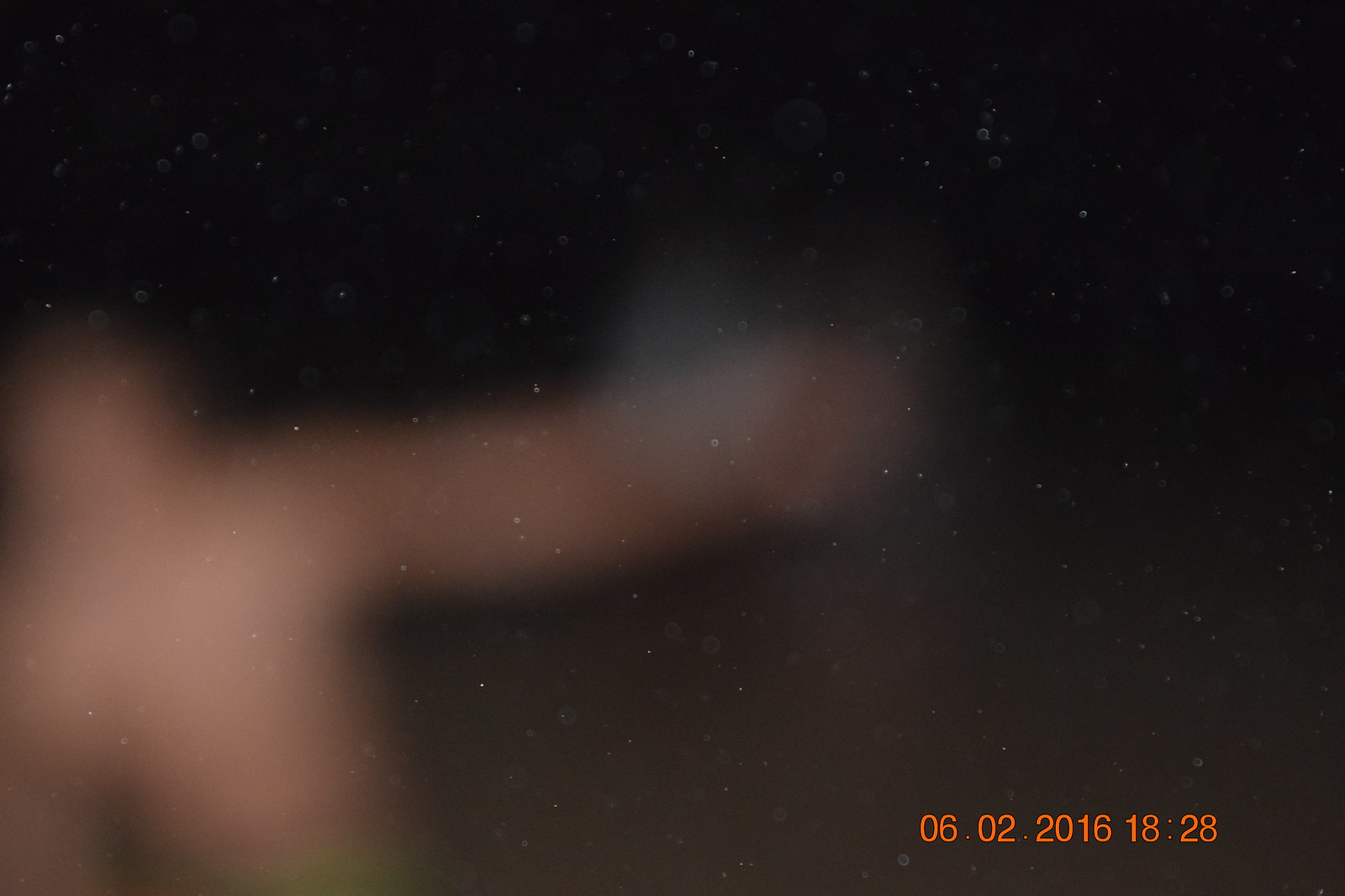The image is a dark and blurry scene, seemingly captured through a pane of glass speckled with dried water droplets. The predominant portion of the image is engulfed in blackness, which appears to depict a night sky. Below this expanse, a brownish strip forms a faint horizon. Emerging from the left-hand side of the frame, there is a vague silhouette of a shirtless person. This figure extends an arm towards the right side of the image, their gesture frozen in the obscured, mysterious ambiance. The indistinct and grainy quality of the photograph, coupled with the natural imperfections on the glass, lends an enigmatic atmosphere to the scene.